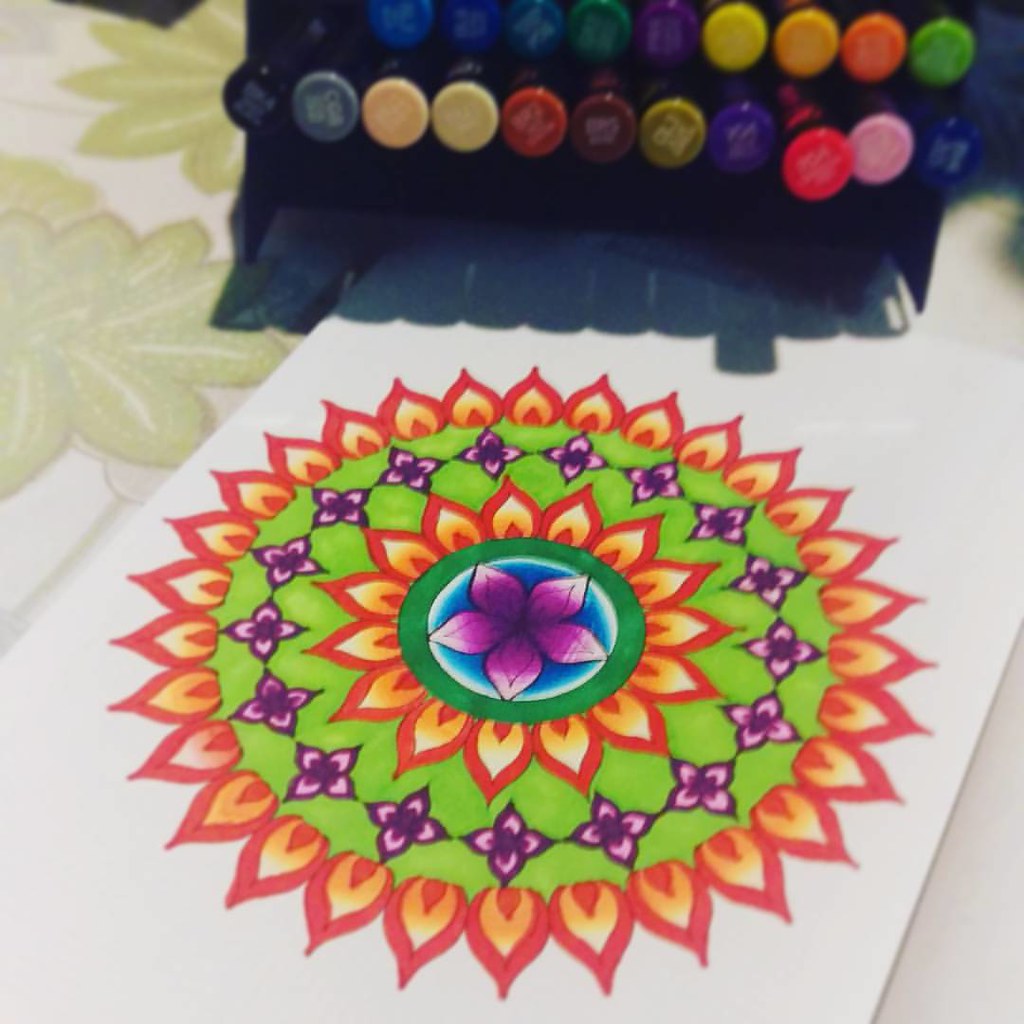This photograph captures an artist's workstation, featuring a white piece of paper adorned with a vivid, marker-drawn mandala. The mandala boasts a detailed, geometric design with a circular, sun-like outer edge made up of yellow and orange flames. Moving inward, lime green shading sets the background for a series of interconnected purple flowers that form a large ring. The next layer replicates the flame motif with orange and red tones, framing another green circle. At the center, a purple flower with blue accents stands prominently, resembling a lotus. Surrounding the paper, various colored markers—including shades of blue, green, purple, yellow, orange, red, and several neutral hues such as gray, black, and cream—are neatly laid out, highlighting the artist's diverse palette. The tablecloth under the art station features a green leaf design, while additional jars of paint in similar vibrant colors are displayed above the artwork.